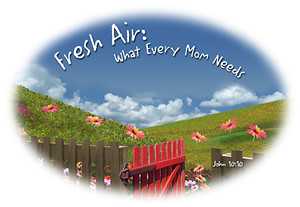The image is an inspiration meme, featuring an oval-shaped scene with a white faded background around it, giving the impression of tunnel vision. At the top edge of the oval, curved text in white reads "Fresh air, what every mom needs." The scene within the oval depicts a peaceful field of grass in a small valley, with blue skies and white clouds overhead. Central to the image is a wooden garden fence with an open red gate, revealing a lush landscape of grass hills and flowers. Among the flowers, six stand taller than the fence, resembling dandelions in bloom. Additionally, the phrase "John 1010" is carved in white into the wooden panel of the fence. This meme, meant to convey a positive and restful message, is designed to be shared over social media.